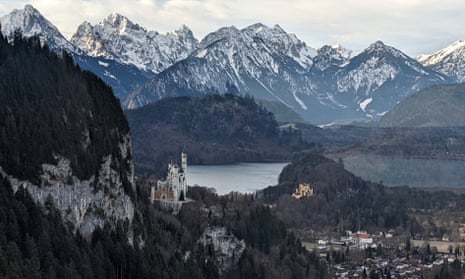This aerial photograph captures a breathtaking view of a vast mountain range, showcasing towering snow-capped peaks in the background with snow cascading down their slopes. Dominating the center of the image is a serene, dark blue lake nestled amid rolling forested hills and mountains. To the left, a sheer cliff face adorned with dark olive green pines descends towards the lake. In the distance, near the lake's edge, a grand castle-like structure with two white spires and a red building at its base stands tall on a hill. This castle overlooks a quaint village situated in a valley towards the lake's base, characterized by small white and tan buildings, many with red roofs. The photograph is bathed in daylight, illuminating the rich green of the trees and the varying shades of brown and white on the mountains and hills.